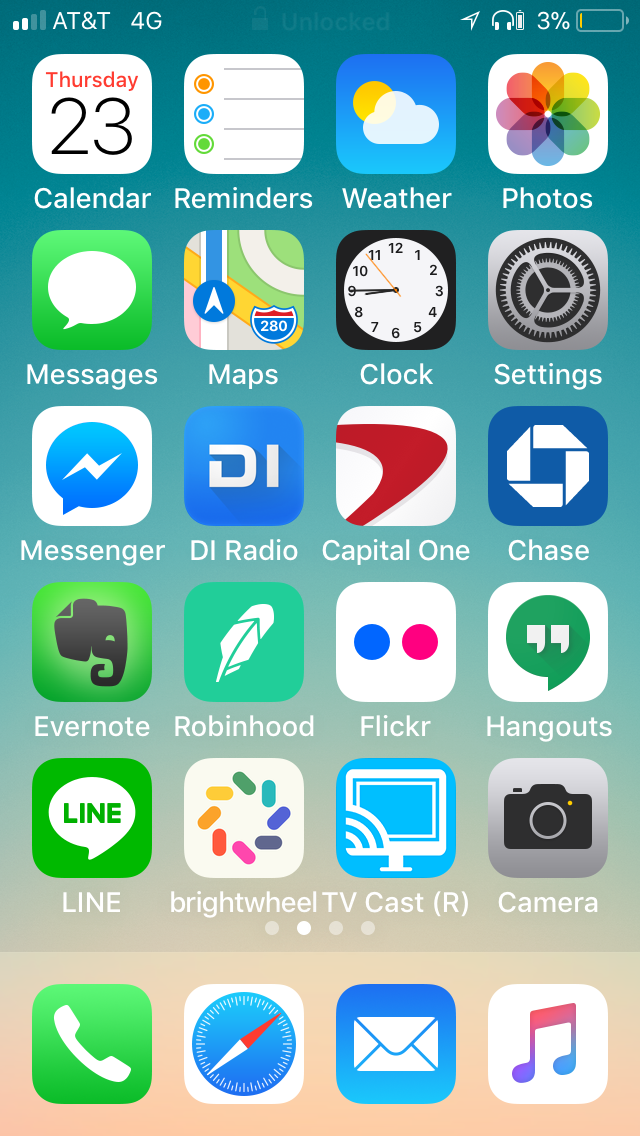The image depicts a highly organized and colorful smartphone screen, filled to capacity with various app icons. The screen utilizes every available space, presenting a vibrant and engaging display. The background transitions from teal at the top to a taupe-like tan at the bottom via shades of light blue and bluish gray. 

In the upper-left corner, signal bars are visible, showing 2 out of 4 or 5 bars, alongside the text "AT&T 4G" in white font. The upper-right corner reveals a battery indicator at a concerning 3%, accompanied by a headphone icon and a directional arrow icon. 

There are six rows of vividly colorful app icons, each row presenting various hues such as lime green, bright blue, and light blue. Notable icons include the multicolored flower of the Photos app and the Flickr app's white background with a blue and pink dot. The overall arrangement gives a festive appearance.

**First Row:**
- Calendar: Displays "Thursday 23."
- Reminders
- Weather: Features a blue box with a cloud and a yellow sun.
- Photos

**Second Row:**
- Messages
- Maps
- Clock
- Settings: Displays a realistic gear image.

**Third Row:**
- Messenger
- DI Radio
- Capital One: Red swoosh.
- Chase: Blue logo.

**Fourth Row:**
- Evernote: Green background with an elephant head.
- Robinhood: Feather icon on an aqua background.
- Flickr
- Hangouts: Speech bubble with quotation marks.

**Fifth Row:**
- Line: Lime green background with "LINE" in a speech bubble.
- Brightwheel: White background with a rainbow circle resembling cupcake sprinkles.
- TV Cast: Monitor icon on a bright blue background.
- Camera

**Bottom Row:**
- Standard icons for Phone, Directional, Email, and Music.

Each row and icon contribute to a cohesive, colorful, and well-organized visual presentation on this heavily utilized smartphone screen, despite some minor connectivity and battery challenges.